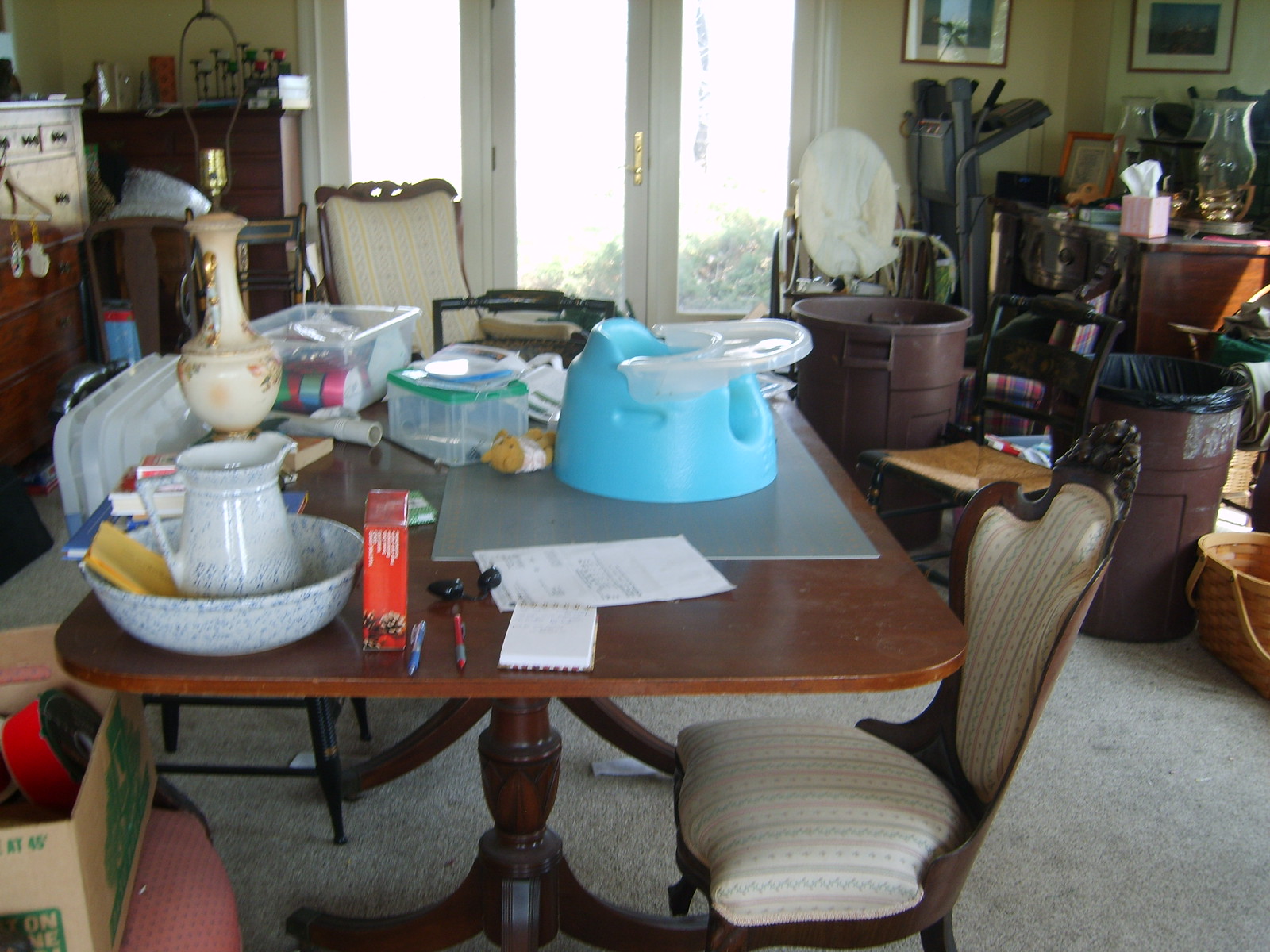The photograph captures a very cluttered living room or dining room, featuring a light tan carpeted floor and yellow walls. The composition centers around three French doors that offer a glimpse of outdoor greenery and a bright, white sky. Dominating the space is a brown wooden dining room table, surrounded by mismatched chairs adorned with various tan patterned cushions. The table is strewn with an array of items including a bowl, a pitcher, boxes, papers, Tupperware, and assorted storage containers. Toys and additional cardboard boxes filled with miscellaneous materials add to the disarray. To the left of the image, two brown wooden armoires stand side by side. On the right, the room becomes even more congested with items such as a folded-up treadmill, tissue boxes, lamps, more chairs, baskets, boxes, and two large brown trash cans lined with black trash bags. The overall scene is one of disorder and functional chaos.